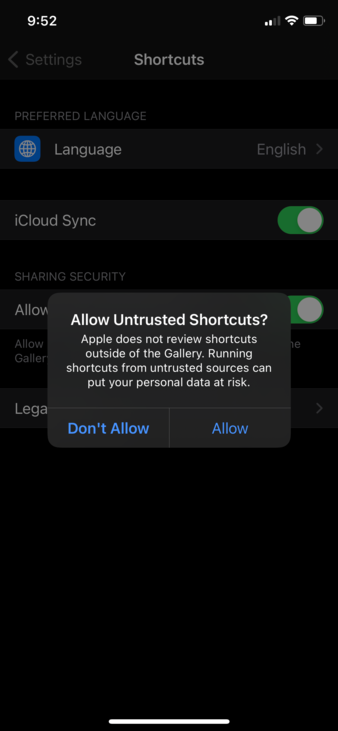A detailed screenshot captured from a phone displays a black background with various system indicators at the top. The current time is shown as 9:52, though it’s unclear if it's a.m. or p.m. To the right, the reception indicator reveals two white bars out of four, indicating weak cellular reception, while the fully white Wi-Fi bars signify a strong Wi-Fi connection. The battery icon is mostly filled, approximately 80% charged.

Below these indicators, the screen header reads "Shortcuts" in white text. Further down, a section labeled "Preferred Language" appears in smaller white font. Adjacent to a blue square icon with a white globe inside, the text "Language" is displayed on the left, while "English" appears on the right.

Next, a section labeled "iCloud Sync" features a toggle switch that is green on the left side and white on the right, indicating the feature is active. Partially visible text mentions "Share and Security," but the detailed content is obscured.

A prominent dark gray pop-up in the center warns about running unverified shortcuts. The alert reads: "Allow Untrusted Shortcuts. Apple does not review shortcuts outside of the gallery. Running shortcuts from untrusted sources can put your personal data at risk." This message is followed by a thin white line, dividing two selectable options: "Don't Allow" in blue on the left, and "Allow" in blue on the right.